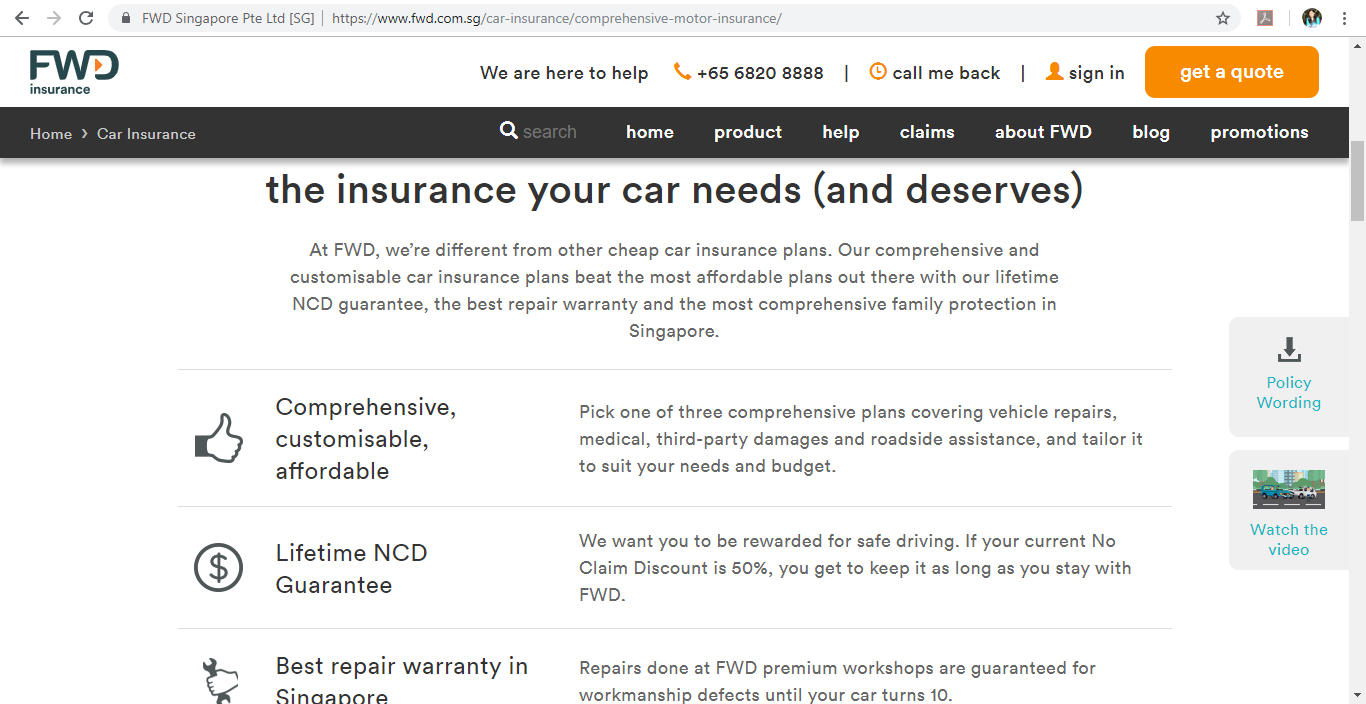FWD Insurance: Comprehensive and Customizable Car Coverage

At the top of the image, "FWD Insurance" is prominently displayed alongside the tagline, "We are here to help." Below this, a phone number is presented with a "Call Me Back" option. Users also have the ability to sign in and request a quote.

A black box underneath lists the covered categories: Home and Car Insurance. The search function is blackened out, and navigation links include Home, Product, Help, Claims, About FWD, Blog, and Promotions.

The main message highlights that FWD Insurance offers superior car insurance designed to meet the needs and expectations of discerning vehicle owners. Unlike other cheap insurance plans, FWD provides comprehensive and customizable plans that stand out due to their lifetime No Claim Discount (NCD) guarantee, the best repair warranty in Singapore, and extensive family protection.

Key features include three comprehensive plans covering vehicle repairs, medical expenses, third-party damages, and roadside assistance. The plans are customizable to fit individual needs and budgets.

Key highlights:
- **Lifetime NCD Guarantee**: Safe driving is rewarded. Retain a 50% No Claim Discount as long as you stay with FWD.
- **Best Repair Warranty in Singapore**: Repairs conducted at FWD premium workshops are guaranteed against workmanship defects until your car turns 10.

FWD Insurance ensures the coverage your car needs and deserves, merging comprehensibility, comprehensive care, and affordability, tailored specifically for the Singaporean market.